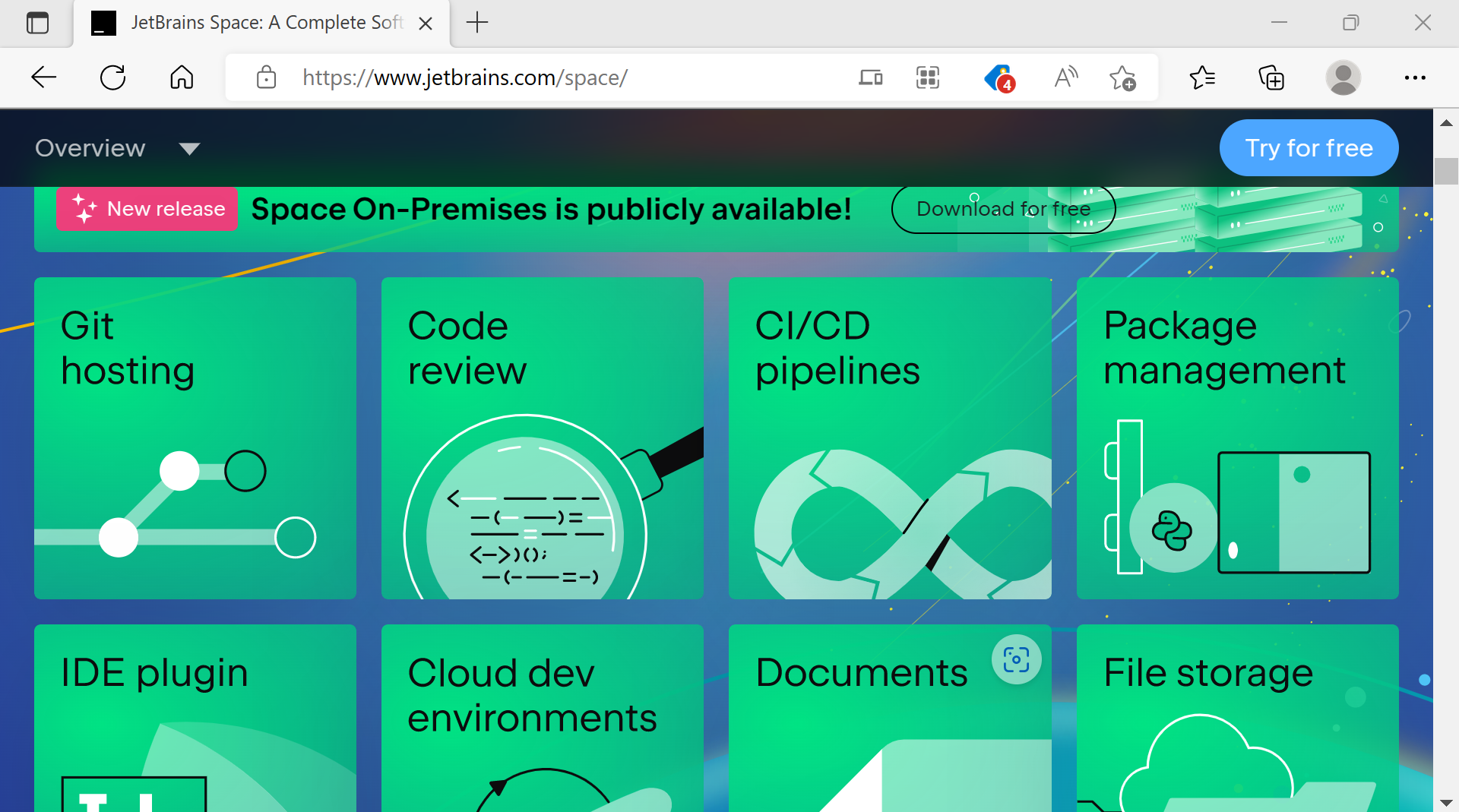A screenshot of a Google Chrome browser on the JetBrains Space website showcases the 'Overview' page. At the top, a prominent banner announces the new release of "Space On-Premises" with the text: "Download for Free." Below this, the main content is divided into eight tiles, each representing a key feature of JetBrains Space: 

1. **Git Hosting** - Illustrated with an icon resembling a map.
2. **Code Review** - Displayed alongside icons featuring dashes, formulas, and a magnifying glass.
3. **CI/CD Pipelines** - Depicted with a figure-eight symbol.
4. **Package Management** - Accompanied by various small icons.
5. **IDE Plugin**
6. **Cloud Dev Environments**
7. **Documents**
8. **File Storage** - Represented by a cloud icon.

The latter four tiles are partially cut off in the screenshot. Additionally, there are four notifications visible at the top-right corner of the browser. The browser tab shows the title "JetBrains Space: A complete", though the full title is truncated. This is the only tab open in the browser window.